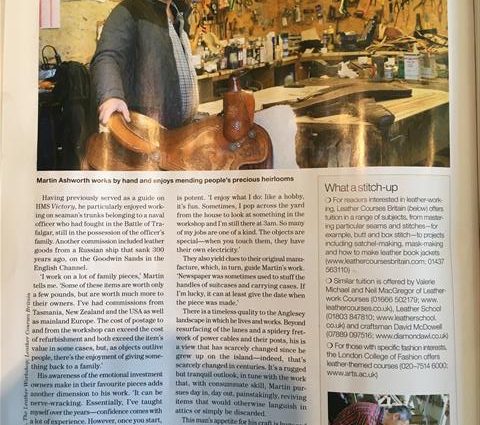This magazine article features an image at the top depicting a man whose face is obscured, but his body is partially visible. He is dressed in a coat and has one hand resting on what appears to be a wooden carving. The background reveals a workbench and a wall filled with an array of tools hanging on what looks like a wooden or cork board.

Below the image, the article discusses Martin Ashworth, a craftsman who specializes in working by hand to mend people's cherished heirlooms. The highligh includes his past experiences serving as a guide on the HMS Victory and highlights his fondness for restoring items such as seamen's trunks, specifically those belonging to naval officers who participated in the Battle of Trafalgar. These heirlooms are still owned by the officers' descendants.

Additionally, on the right side of the article, there's a highlighted section titled "What a Stitch-Up," accompanied by bullet points. There is also a smaller image in the bottom right corner of another man. The details of the article are somewhat challenging to discern due to the low resolution of the image.